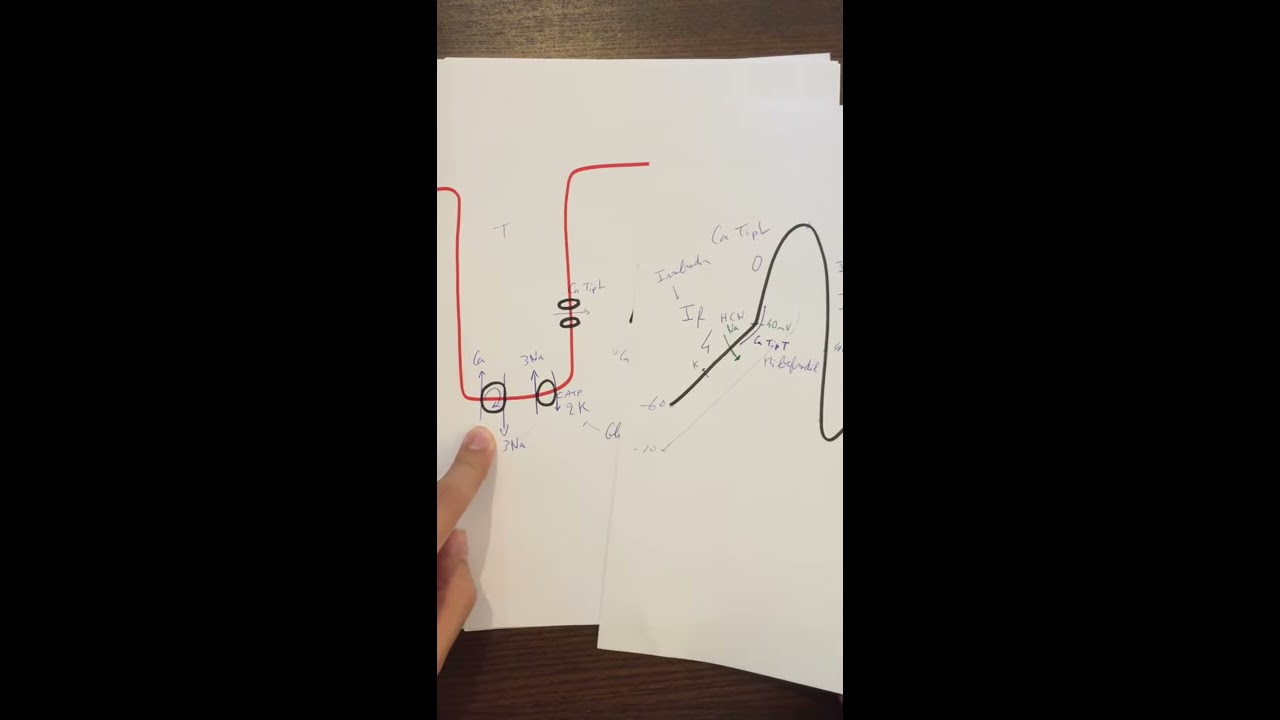In this close-up image, a stack of white papers rests on a dark brown wooden table. Dominating the center of the image is a prominently placed stack of paper, partially overlaid on the right by another sheet. On the left side of the central paper, there is an index finger pointing towards a red loop-shaped diagram—reminiscent of a U-shape—embellished with four black circles and accompanying numbers. The diagram looks intricate, suggesting it could be related to an electrical circuit or similar technical subject matter. Meanwhile, the overlaid paper on the right features a bold black line that ascends, curves, and descends again, accompanied by various handwritten letters, numbers, and symbols. The image dimensions suggest it might be a still from a portrait-framed video, with black bars on either side framing the central composition.